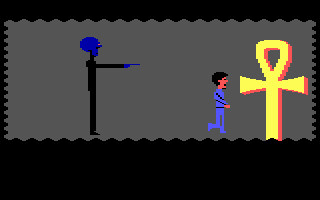The image depicts a scene reminiscent of a video game environment. The background is a deep, jet-black with no visible texture or gradient, providing a stark contrast to the central elements. Dominating the scene is a wavy gray rectangle with undulating edges, featuring smaller waves on the sides and larger ones on the top and bottom.

In the foreground stands a slender character, stylized in the manner of a video game avatar. This character is dressed entirely in blue - from the top to the pants - and sports black hair. A notable feature is the character's blue head, enhancing its otherworldly appearance. The character appears to be pointing either a blue finger or a weapon towards a small child nearby.

Adjacent to this character is a yellow cross, framed subtly in orange, adding to the scene's rich visual narrative and hinting at potential interactions or objectives within the game.